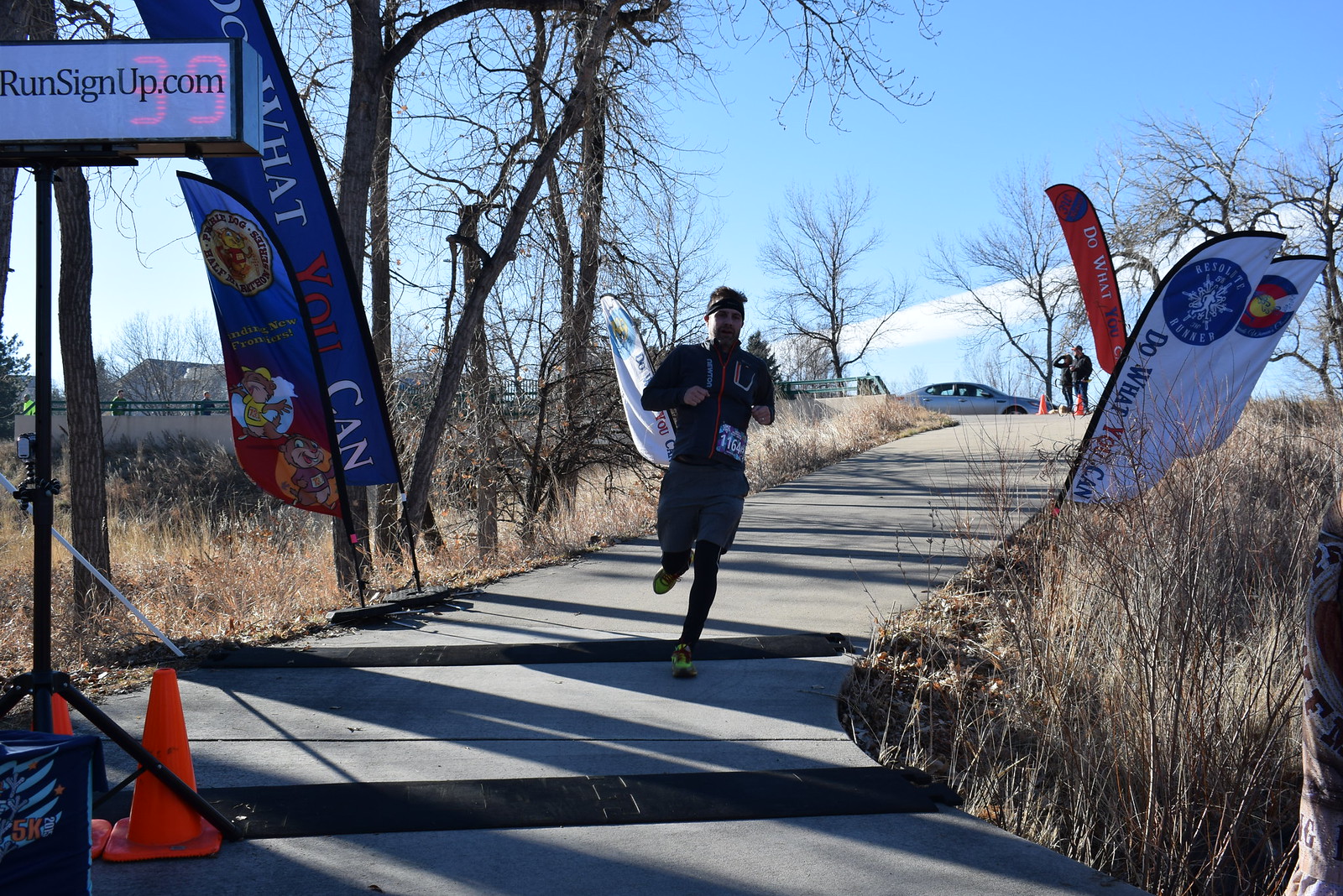The photograph depicts a dynamic scene of a runner competing in a footrace, set on a concrete sidewalk that cuts through a wintery or early spring landscape characterized by barren trees and gray, leafless shrubbery. The runner, dressed in a dark jersey, gray shorts, white stockings, and yellow-green shoes, is captured in mid-stride, advancing towards the camera. He has just crossed over a black rubber strip on the sidewalk and is about to cross another, near an orange caution cone positioned in the lower left corner of the frame. Lining both sides of the path are various colorful banners and flags—blue, red, and white—each adorned with symbols or motivational phrases like "do what you can," and serving as advertisements, with one prominently displaying "runsignup.com" alongside a digital number "39." The sky overhead is a light blue with scattered clouds. In the upper background, to the right of the path, stand two individuals next to a parked car, observing the race, contributing to the organized and monitored atmosphere of the event.